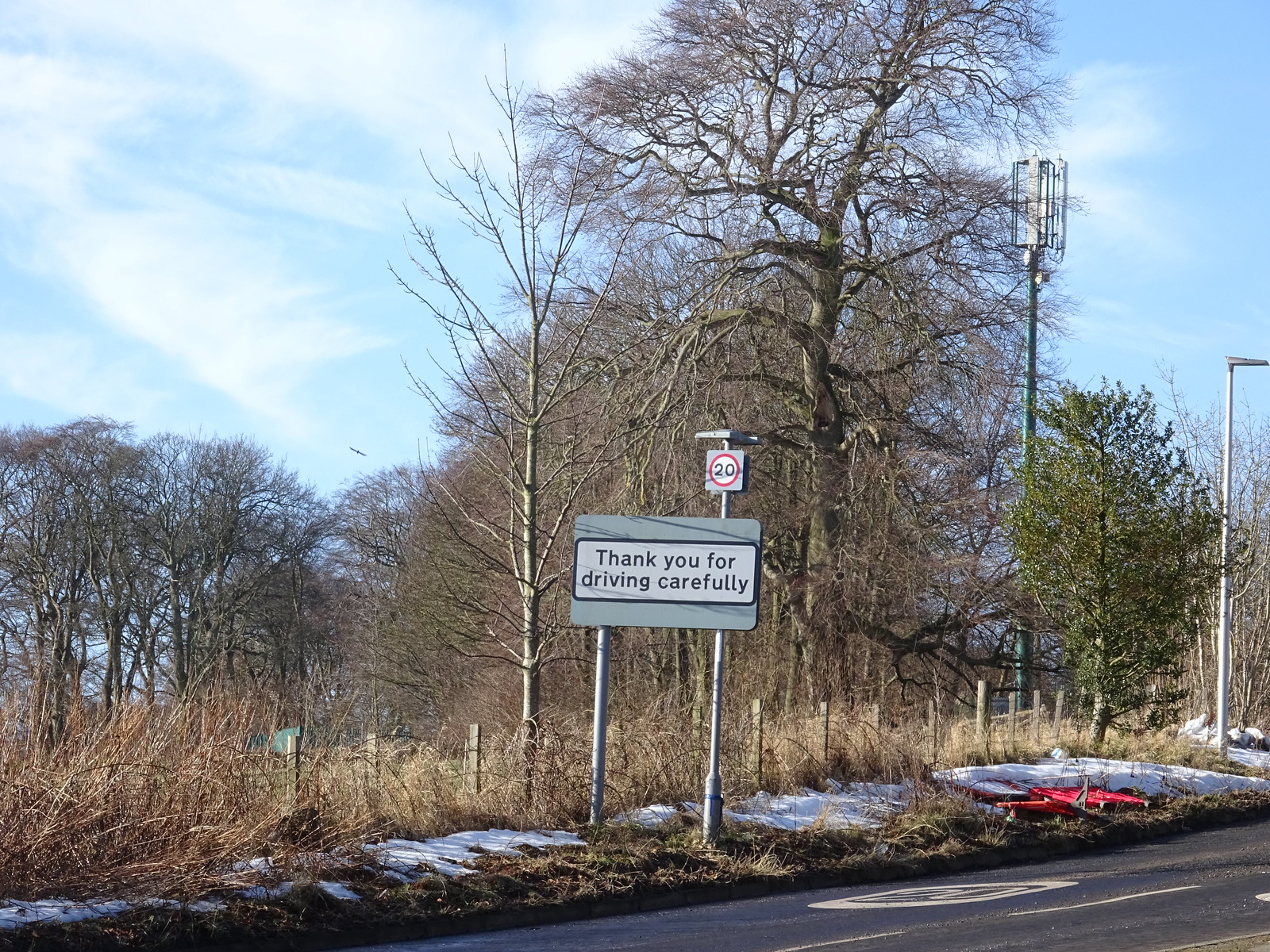The image depicts a rural roadside scene under a partly cloudy yet predominantly blue sky, creating a serene winter atmosphere. A road with dark gray concrete and yellow center stripes stretches diagonally from the bottom middle toward the upper right. Flanking the road is mowed green grass, while on the other side of an old wooden and wire fence, taller brownish vegetation and patches of snow are visible. The fence, composed of aged wooden posts and cables, demarcates the transition from the maintained grass to the wild, untamed area. Trees, mostly bare due to the winter season, frame the background, with a lone evergreen standing out amidst its leafless counterparts.

At the heart of this scene, a sign stands prominently near the roadside, affixed to two silver poles. The green, horizontal rectangular sign, framed by green letterboxes at the top and bottom with black text in the center, politely reads, “Thank you for driving carefully.” Above this sign, a smaller speed limit sign, possibly indicating 20 miles per hour, is barely visible. The juxtaposition of the bare trees, scattered snow, and clear signage encapsulates the quiet, contemplative essence of a rural winter's day.